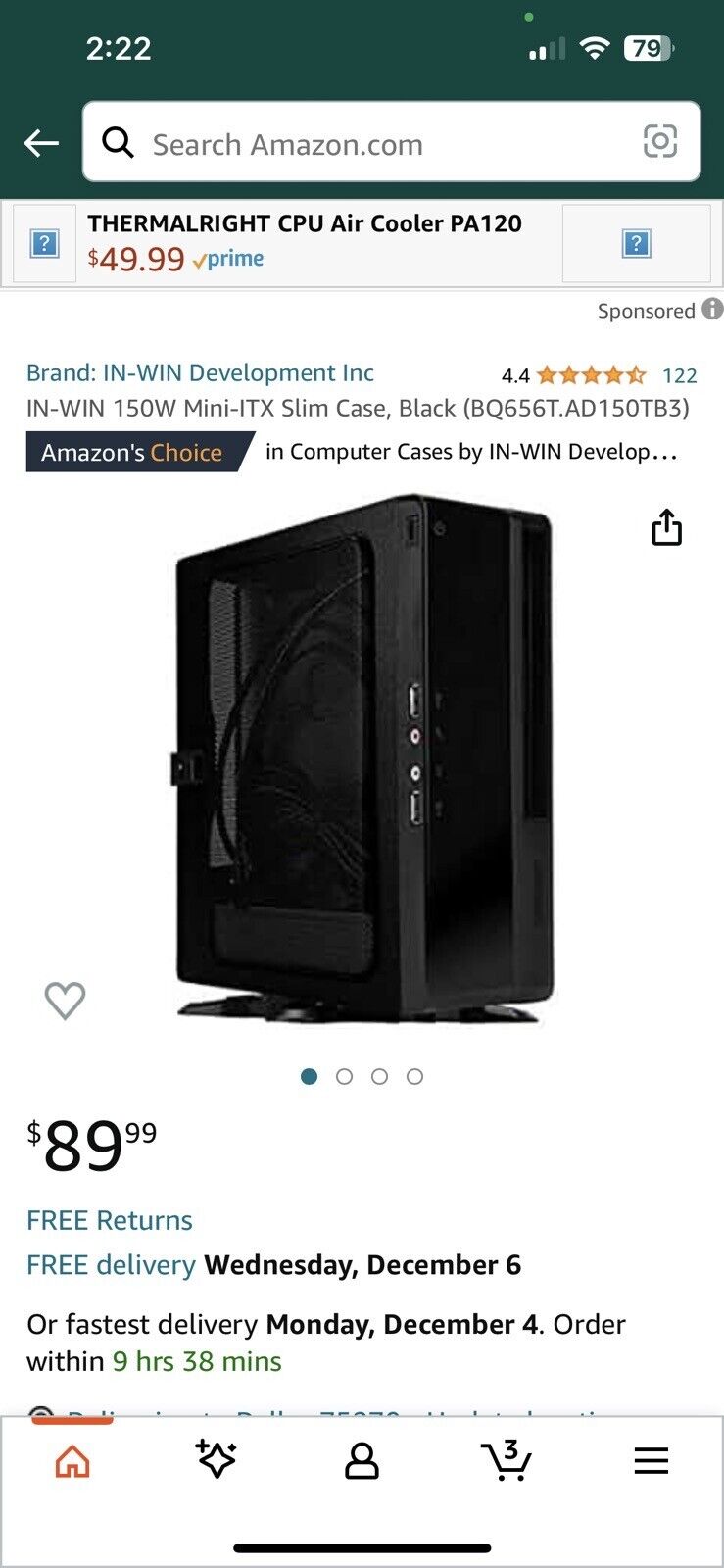Screenshot of the Amazon Shopping App

The displayed screenshot captures a detailed view of the Amazon Shopping app, specifically focusing on a product page. The top title bar of the app is green, and the status indicators reveal that the screenshot was taken at 2:22 PM with a battery charge of 79%. Below the title bar, there is a search bar labeled "Search Amazon."

The main content area of the screenshot showcases the product page for a Thermalright CPU Air Cooler PA120, priced at $49.99 and available as an Amazon Prime deal. The brand is NWIN Development Incorporated. Following this, details for another product, the NWIN 150W Mini ITX Slim Case in black, are presented. The product ID for this case is BQ656T.AD150TB3, and it is highlighted as an "Amazon's Choice" in computer cases by NWIN Development.

Displayed prominently on the page is a picture of the desktop tower, which is entirely black with a few white buttons. The listed price for this case is $89.99, with benefits including free returns and free delivery by Wednesday, December 6th. Additionally, it mentions an expedited delivery option by Monday, December 4th, if ordered within 9 hours and 38 minutes from the time shown in the screenshot.

Finally, the bottom toolbar of the Amazon app is visible, featuring icons for the Home, Account, Shopping Cart, and Menu buttons.